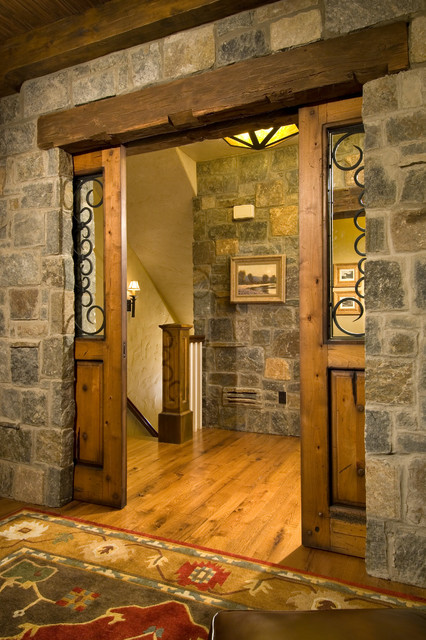The image showcases a rustic, elegant doorway leading into a room adorned with intricate details and rich textures. The doorway features two tan brown wooden pocket doors with visible knots, complemented by subtle metallic swirls within the glass panes. These doors sit within a robust frame of dark wood and are set into walls made of gray and brown stone, hinting at an old building’s solid and timeless architecture. 

On the hardwood floor at the entrance, a vibrant Persian or Oriental rug with yellow, blue, red, white, and black floral designs adds a splash of color and sophistication. Just beyond the doors, a stairway ascends to the left, with a yellow, rustic-style ceiling light overhead and a sconce light on the stairwell wall. Directly through the doors, a small painting depicting trees and a body of water, perhaps a lake or pond, draws the eye. To the right, additional framed pictures adorn the yellowish stone wall. A barely visible dark brown ottoman or sofa leg also adds to the room's cozy, eclectic aesthetic.